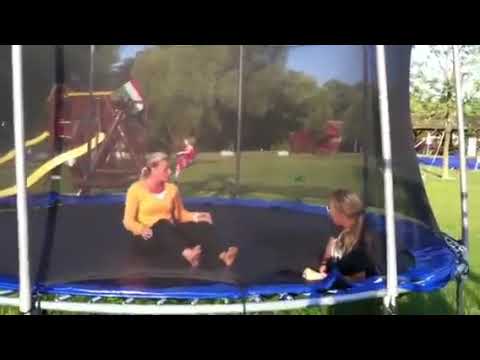In this photo, taken on a bright, sunny day at a playground, two blonde women in their twenties sit barefoot on a screened trampoline, deeply engaged in conversation. The woman on the left wears a yellow sweater with black pants and is animatedly moving her hands as she talks. The woman on the right, dressed in a black sweater, listens intently. Surrounding the trampoline, the playground features a swing set in the background where a child in a red outfit is joyfully swinging. The area is lush with green grass and flanked by trees, creating an inviting scene for recreational activities.